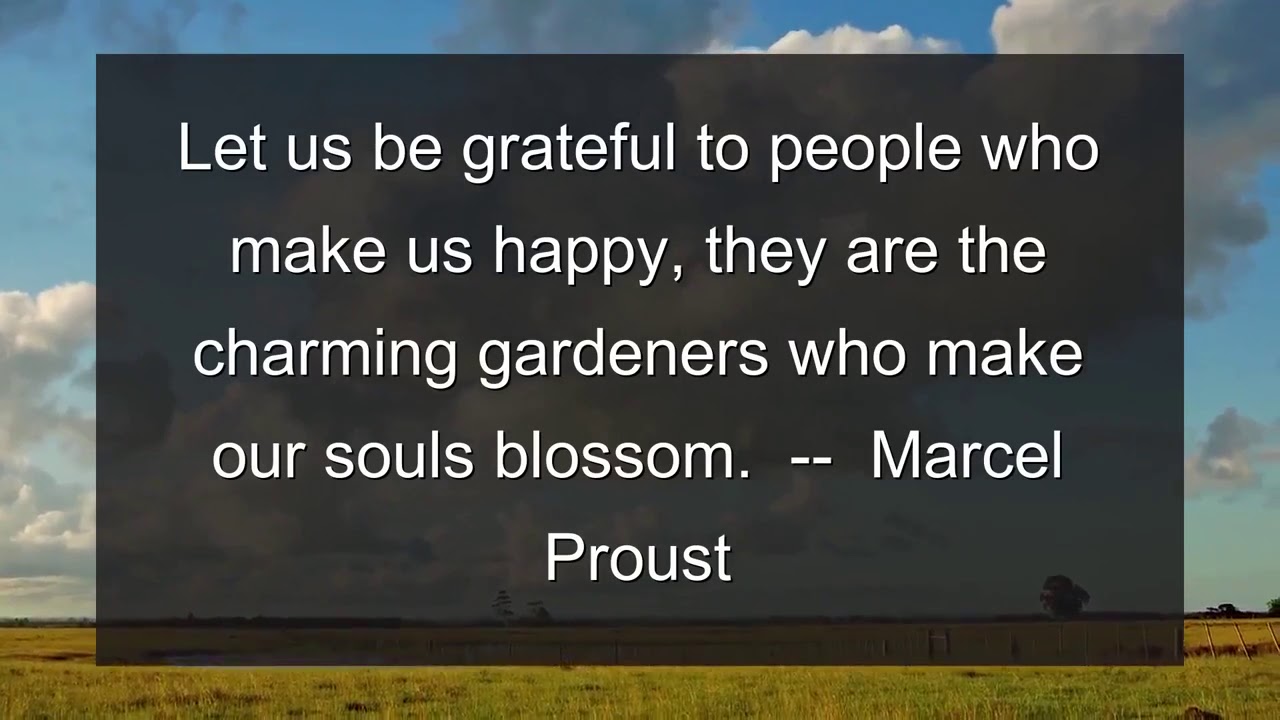In this image, a profound quote by Marcel Proust is elegantly presented in white text on a semi-transparent, charcoal gray rectangular box. The text reads, "Let us be grateful to people who make us happy; they are the charming gardeners who make our souls blossom." The transparent nature of the box allows a beautiful prairie landscape to show through, comprising vibrant green and yellow grasses, indicative of an arid region. Scattered wooden posts suggest the presence of a fence line. Above this sprawling field, the sky shifts from deep blue at the top to lighter shades near the horizon, adorned with thick, billowing cumulonimbus clouds. The harmonious blend of the poignant quote and the serene, open field background creates a visually and emotionally compelling image.